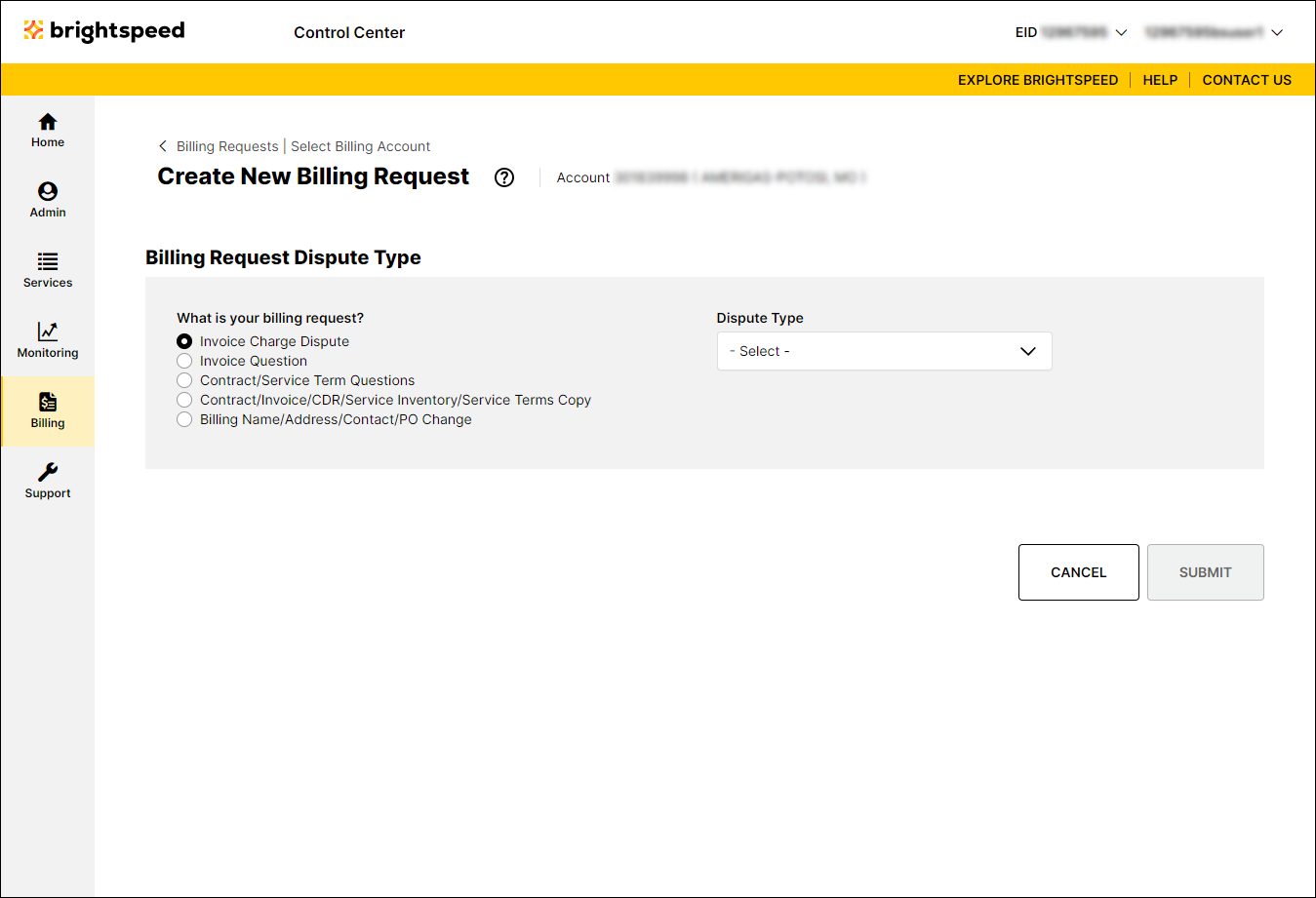This image displays a detailed view of the Brightspeed Control Center web page. The page prominently features a navigation menu with various links such as "Explore Brightspeed," "Help," and "Contact Us." Categories listed include "Home," "Admin," "Services," "Monitoring," "Billing," and "Support."

Under the "Billing" category, users can find options like "Billing Requests," "Select Billing Account," and "Create New Billing Request." There are specific billing request types available such as "Invoice Charge Dispute," "Invoice Question," "Contract Service Term Questions," "Contract Invoice CDR," "Service Inventory," and "Service Terms Copy." The form further requires details such as "Billing Name," "Address," "Contact," and "P.O." 

This comprehensive web interface is designed to facilitate various customer inquiries and service management related to Brightspeed.